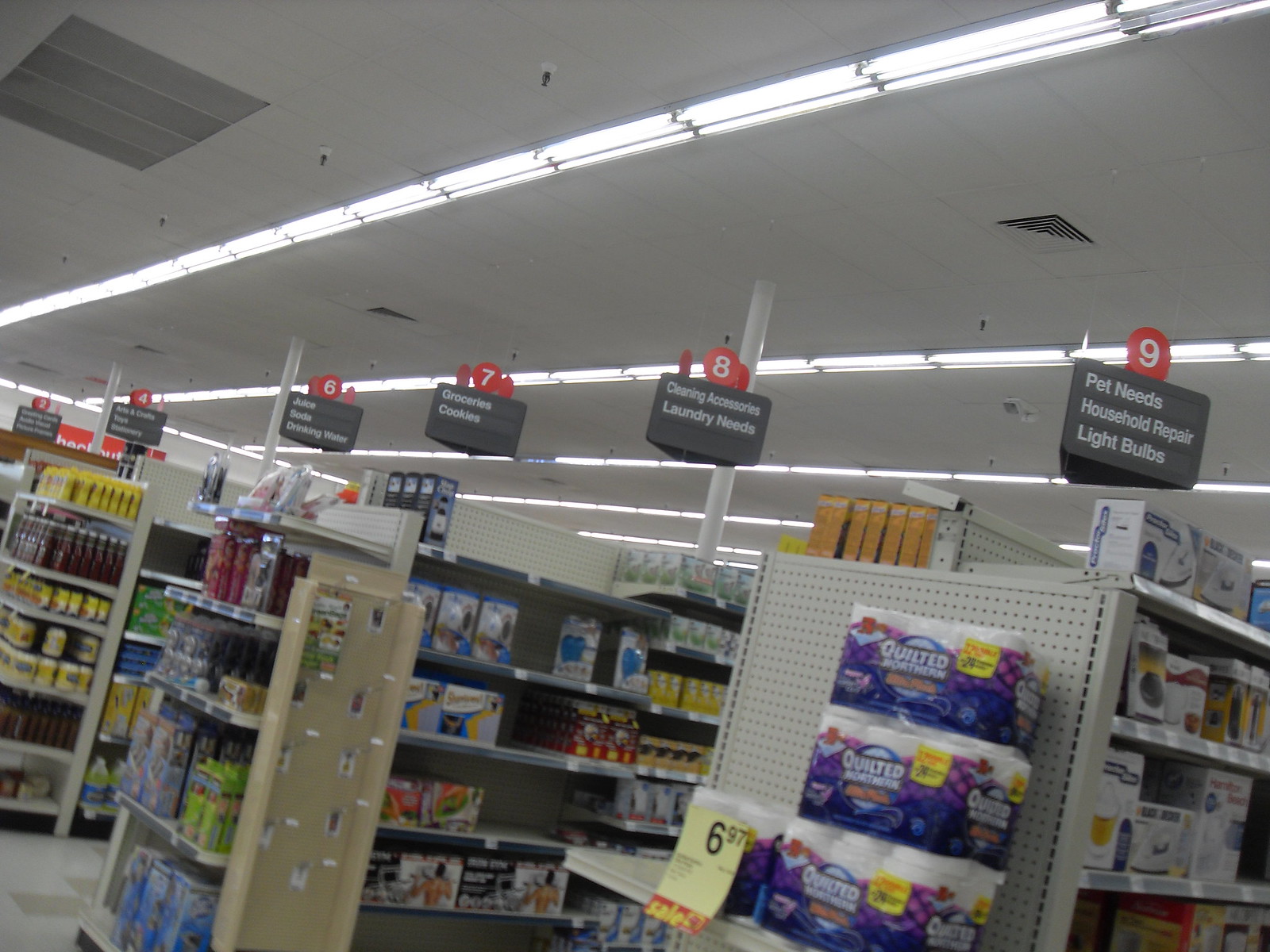The image captures the interior of a store, taken at a slight slant, tilting downward towards the right. This perspective reveals three aisles and the store's ceiling, which displays numbered signs indicating the contents of each aisle. From left to right, nearing the camera on the right side, the aisle numbers visible in the shot are 2, 4, 6, 7, 8, and most prominently, aisle 9. Each aisle is marked by a gray sign hanging from the ceiling, detailing the items found within. Aisle 9 is the most legible and closest to the viewer, standing out more clearly in the scene.